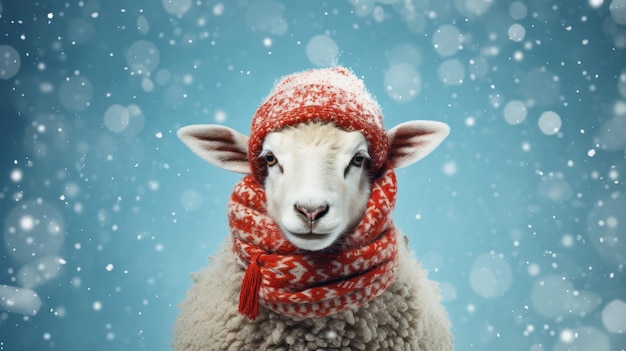This image showcases what appears to be a computer-generated or artistic rendering of an incredibly cute lamb amidst a snowy background. The lamb is centrally positioned against a blueish-white backdrop filled with variously-sized snowflakes, giving a textured, bokeh effect that suggests depth and a gentle snowfall. The lamb's fleece is thick, light-colored with hints of white and beige, some of it appearing to be lightly dusted with snow. Its ears stick out endearingly to the sides, contrasting with the vibrant red knit cap and matching red and white scarf it is wrapped in. The lamb’s face, which features a white and tan coloration, gazes directly into the camera, embodying an innocent and heartwarming expression. The image contains no text, allowing the lamb's adorable presence to stand out beautifully.